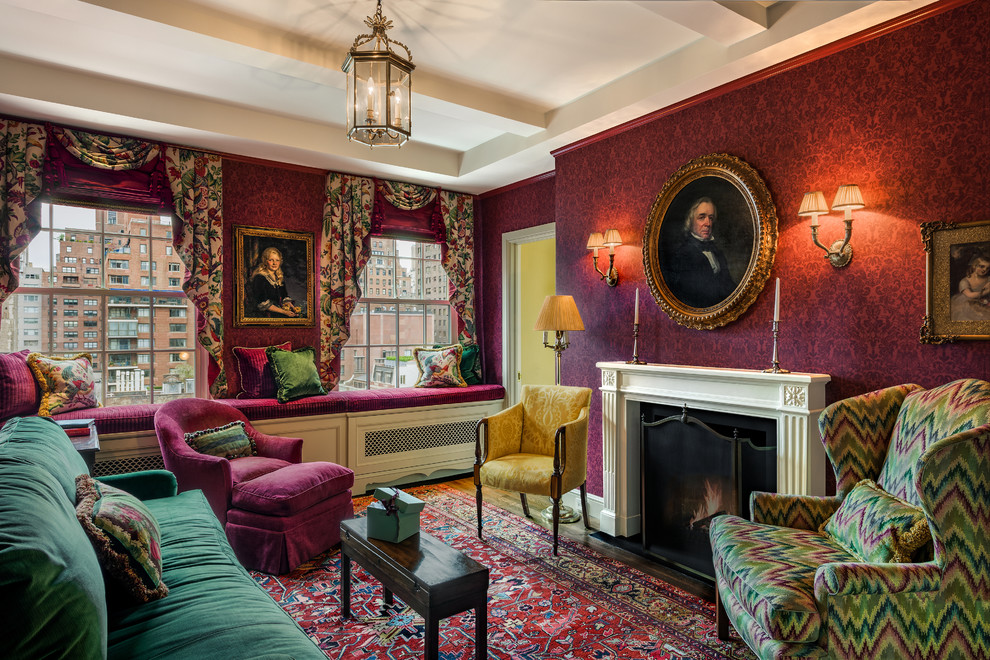The luxurious living room exudes Victorian elegance with its tall, white-beamed ceiling and deep reddish-pink textured wallpaper. Natural light filters through the floral curtains adorning two large windows, which provide a view of an urban cityscape, possibly in Europe. Below the windows, a cozy window seat is lined with plush pink cushions and pillows. The room is anchored by a grand white-columned fireplace, where a fire flickers warmly beneath an ornate gold-framed portrait of a man from the 17th or 18th century. Additional oil paintings, including portraits of a woman and a child in similar opulent frames, adorn the walls, enhancing the room's historical ambiance.

Furniture pieces add both style and comfort to the space, with a yellow armchair beside the fireplace and a red armchair with an ottoman near the window seat. A green sofa with a floral pillow is complemented by a chair featuring a green and pink zigzag pattern. The room's centerpiece, a small coffee table, sits atop an expansive Persian rug that incorporates shades of pink, red, brown, and hints of blue. The decor is further unified by purple-themed accents, including purple sconce lights and a chair with matching seat cushions. Overhead, a chandelier with candle-like lights illuminates the room, completing the picture of opulence and refined taste.